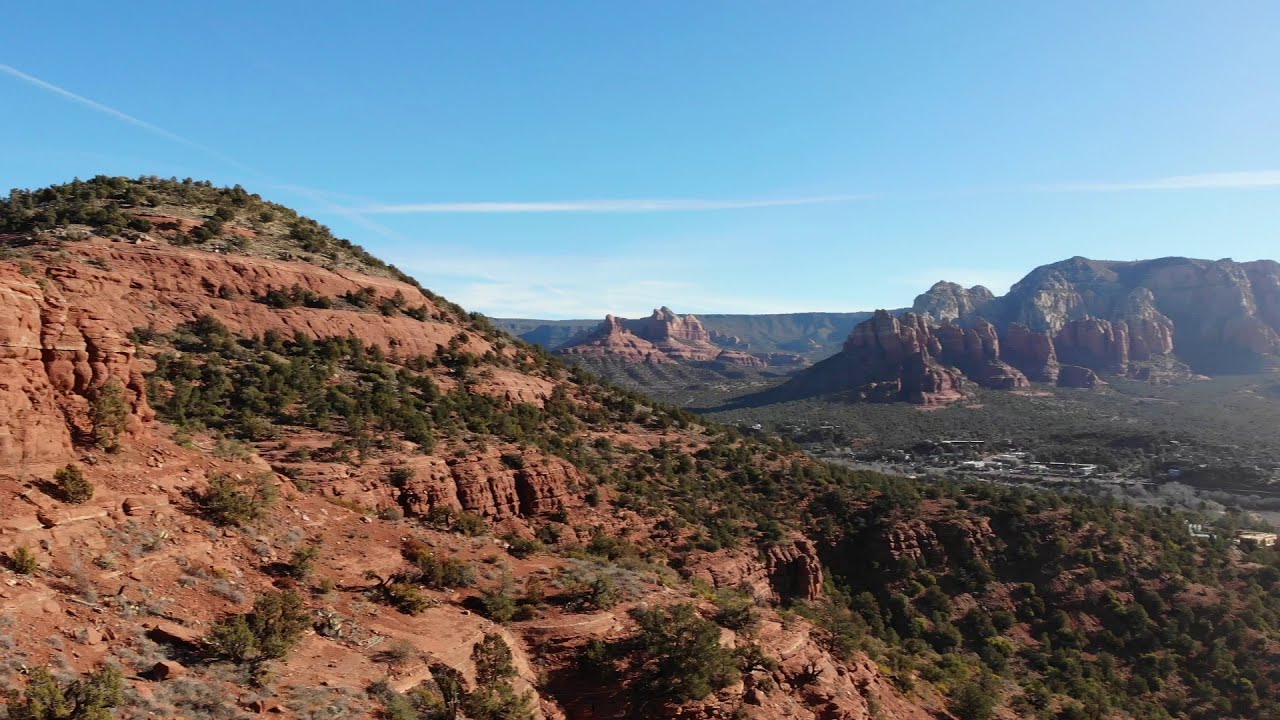This captivating image showcases a vast high desert mountain range, likely in Utah or a nearby region. Dominating the left side for about two-thirds of the photo is a large, rocky red mountain, adorned with sparse greenery and dry brush. The mountain's rugged terrain gradually descends into a flat valley area towards the right, which is dotted with vibrant green grass and a serene hint of water. Nestled in this valley is a small town, complete with building shops and a neighborhood of houses that extend into the picturesque landscape. Beyond the valley and small town, another imposing red cliff stands proudly, mirroring the craggy beauty of the foreground mountain. Further back, a series of smaller mountainous formations stretch towards the horizon, intricately framing the scene. The sky overhead is a brilliant blue, sparsely decorated with thin, wispy white clouds, adding a touch of serenity to this striking desert tableau.